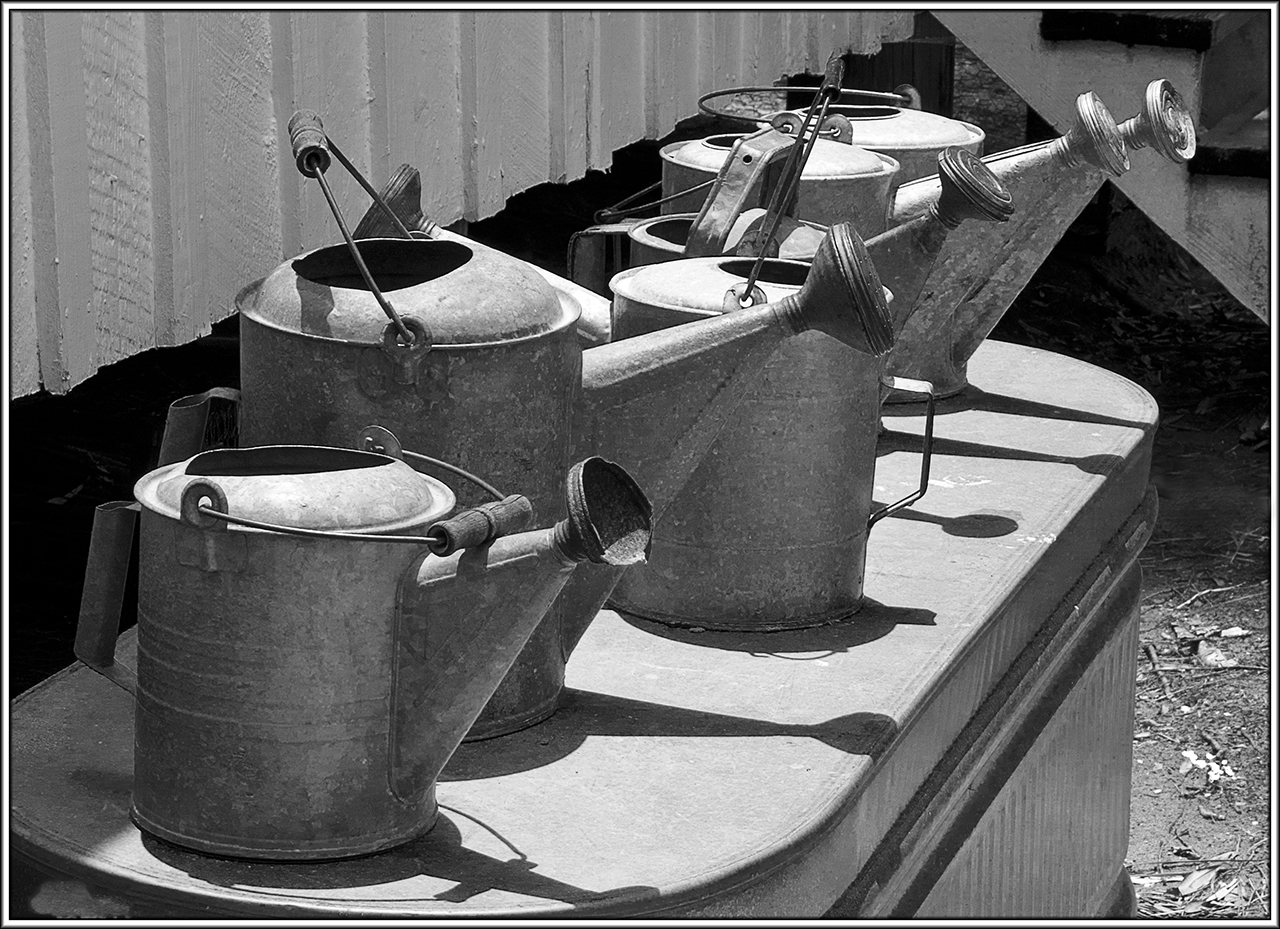This black and white photograph captures a collection of six metallic watering cans, each varying in size and positioned atop a metal container with a rounded rectangular form. The watering cans, appearing slightly aged, are made of a silvery steel and each features a handle on top for carrying, along with a side handle for pouring. Their spouts are elongated with cylindrical sprinkler heads that have perforations for dispersing water. 

Among the cans, one smaller can is in front, followed by a larger one behind it, another smaller one beside the larger can, one turned in the opposite direction, and two more large cans. The background reveals aluminum paneling or white wooden paneling, suggesting part of a building. The image also shows some details of a potential set of stairs with white railings and darker planks in the upper right corner. The ground surrounding the metallic container is scattered with leaves, twigs, and rocks, emphasizing the photograph's grayscale and detailed texture.